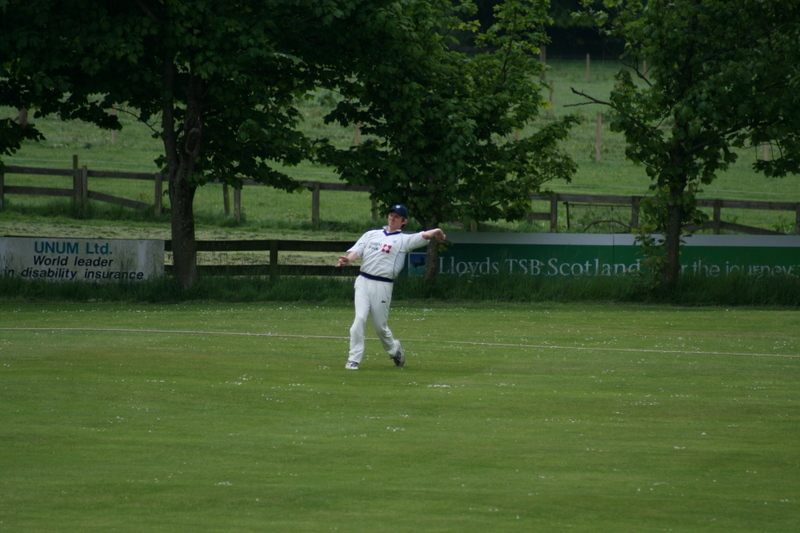This photograph captures a dynamic moment in a lush green field, featuring a baseball player mid-action as he prepares to throw a ball. The athlete wears a white uniform consisting of a shirt, pants, and shoes, complemented by a blue cap. Behind him, the boundary of the field is dotted with trees and lined with advertisements along the wall. Beyond this wall is a wooden fence, and further in the distance, another stretch of vibrant green grass extends into a remote pasture. The scene is a picturesque blend of athletic spirit and serene natural surroundings.